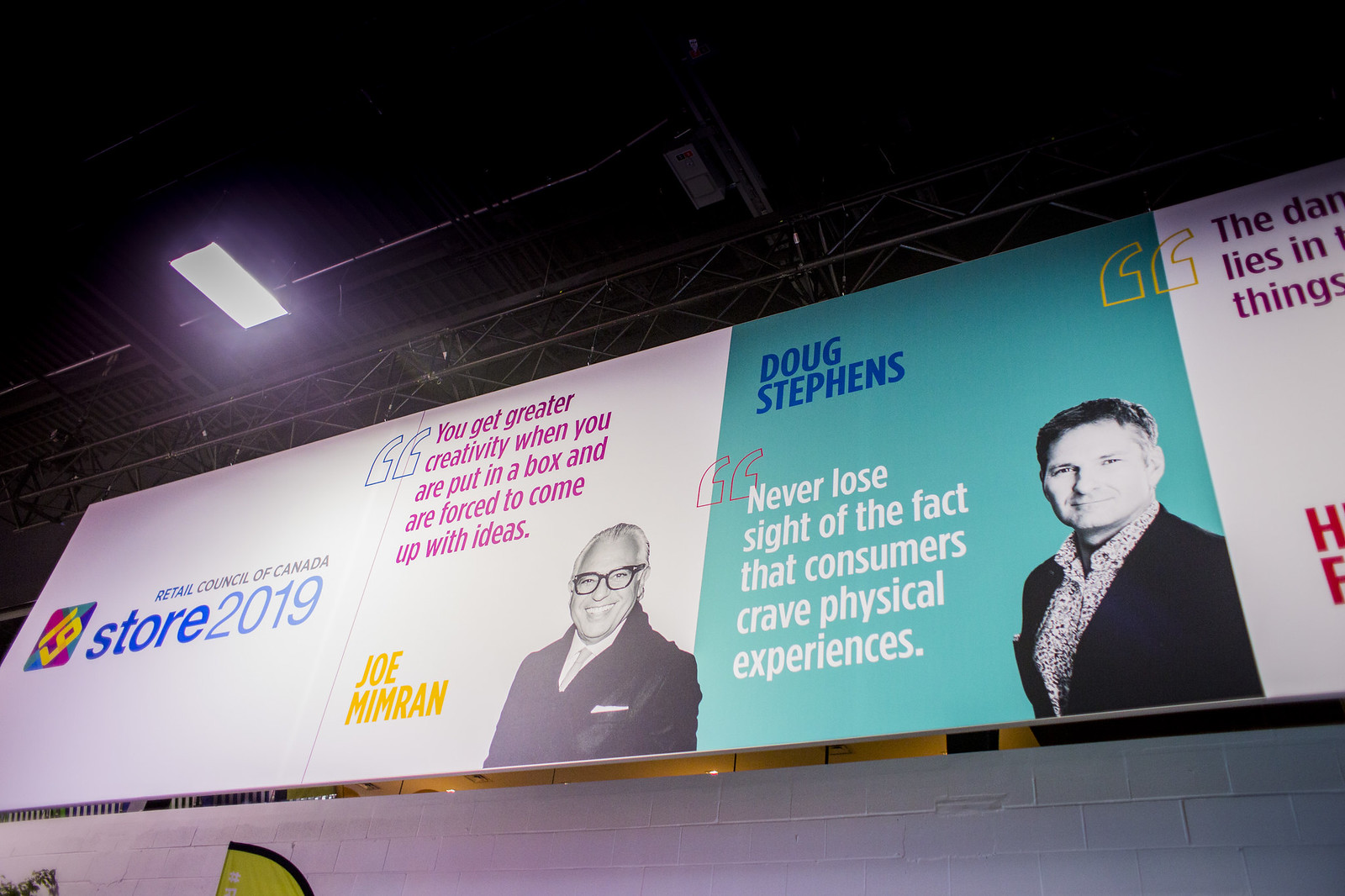The image features a detailed scene centered around a billboard, likely taken in an interior setting, such as a stadium or large hall, though it could be outside at night given the dark surroundings. The billboard is prominently positioned in the center of the image. At the bottom, a rugged brick wall serves as a baseline, adorned by a few indistinct items in the bottom left corner. The top portion of the image displays an off-white roof structure with dim lighting, suggesting an enclosed environment.

The billboard displays a variety of information and visuals. Dominating the center is an advertisement for the "Retail Council of Canada Store 2019," presented in various shades of blue on a white background. The advertisement is quite text-heavy, featuring quotes from Joe Mimron and Doug Stevens. One notable quote reads, "You get greater creativity when you are put in a box and are forced to come up with ideas." The imagery includes a smiling man with glasses, further emphasizing a message about the consumer demand for physical experiences. 

The color palette is diverse, featuring off-white, yellow, black, blue, light blue, purple, red, and yellow hues. Luminescent lights and shadows play across the top, contributing to an overall ambiance that hints at an indoor setting. This complex and textured image captures a dynamic advertising scene rich with contrasting elements and detailed messaging.